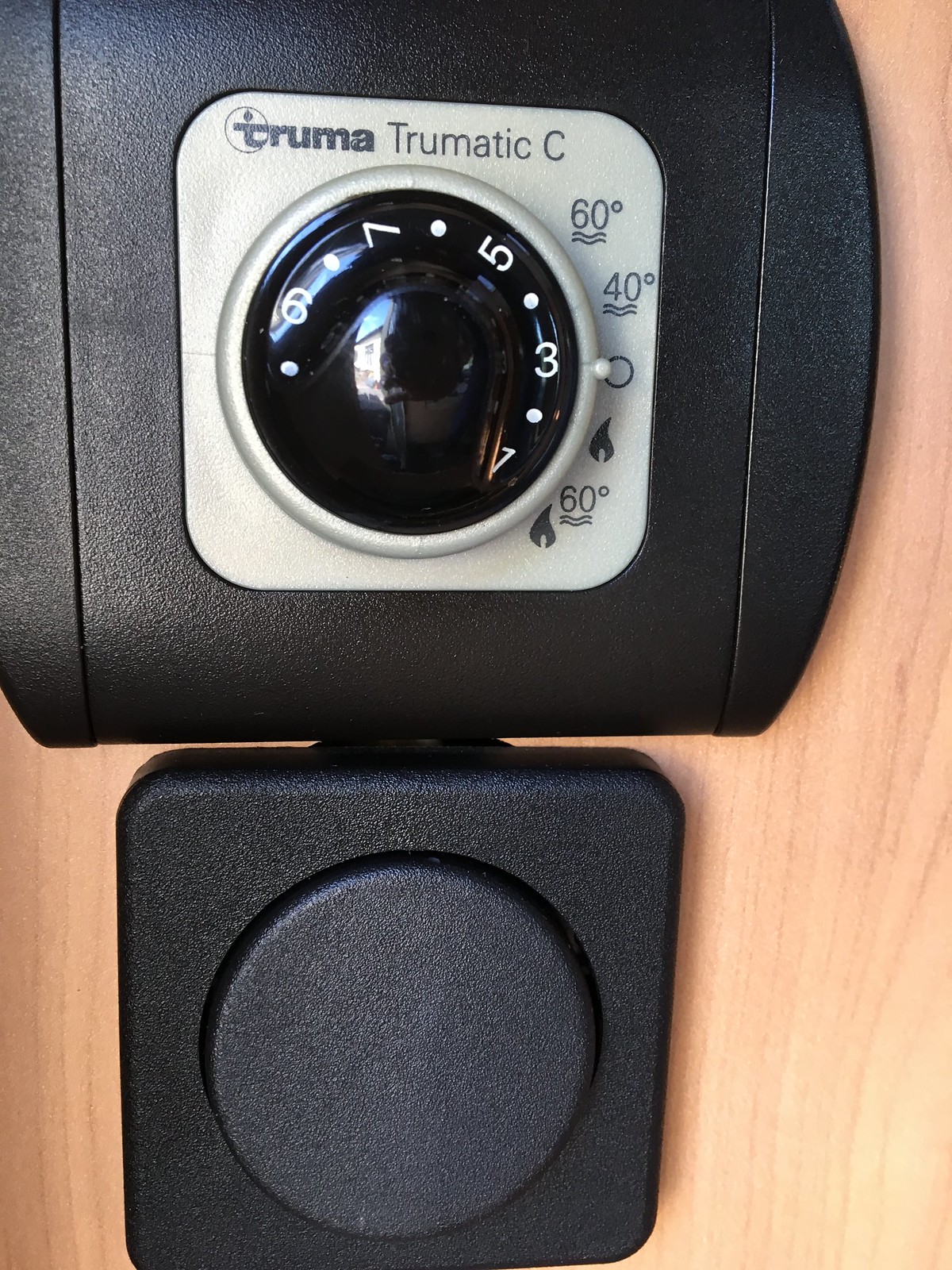The image depicts a wall adorned with light woodgrain paneling, giving off a subtle, natural aesthetic. At the bottom of this wall, there is a black plastic square featuring a circular button in the center, suggesting it might be an interactive element, though its function is unclear.

Mounted above the plastic square is a black thermostat, which includes a sleek silver interface housing a controller. The branding on the device reads "Truma Trumatic C." The temperature settings displayed on the thermostat range from 60 degrees, with additional markings indicating 40 degrees, although only the 60-degree mark is prominently shown, suggesting the measurements are in Celsius. Additionally, there are flame icons indicating heating options. The central knob on the thermostat features increments of 1, 3, 5, 7, and 9, likely representing different levels of temperature or heating intensity.